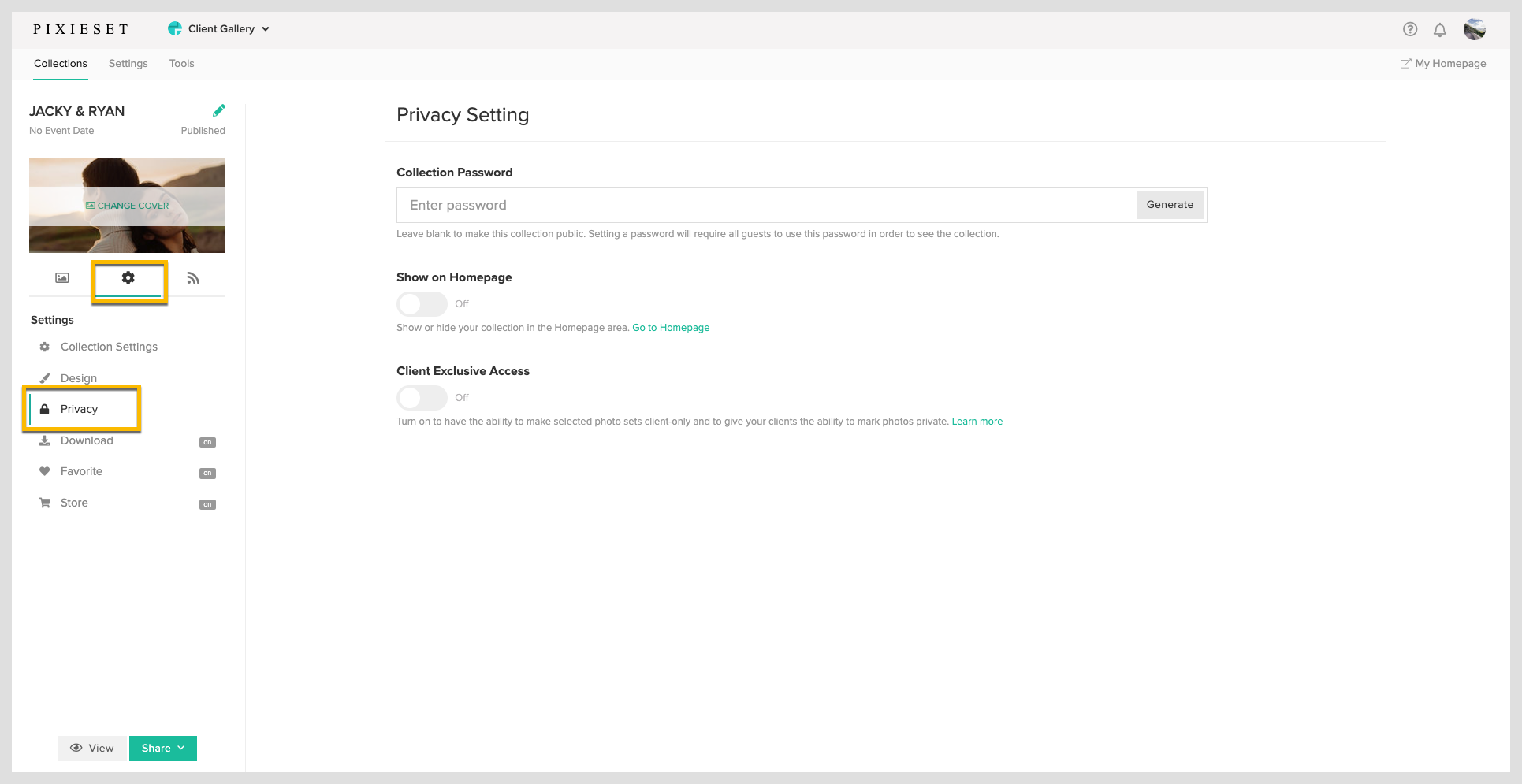The image depicts a white background with a prominently outlined light blue border around the entire box. At the top, there is a blue circle with a checkmark, next to the text "A Pixie Set." Below this, the names "Jackie and Ryan" are displayed, accompanied by a small picture. Adjacent to this picture is a yellow square enclosing a star-like icon. Further down, there is a section labeled "Settings," and to its right, another section labeled "Privacy Settings" with three distinct headings. On the far right side of the image, there is a small blue box. At the very bottom, within the large white box, there is a greenish-colored box that appears to be labeled "Open." The entire content is neatly contained within the light blue outline.